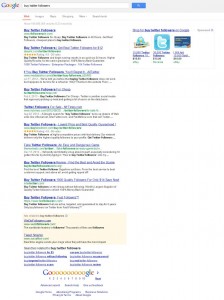The image depicts a blurred Google search results screen displaying approximately 10 listings on a white background. At the top, a gray bar spans across the screen with the Google logo situated on the left side. The Google logo consists of a blue capital 'G', followed by lowercase 'o's in red and yellow, a blue lowercase 'g', a green lowercase 'l', and a red lowercase 'e'. Centered in the gray bar is a white search box containing an illegible three-word query. Adjacent to this search box on the right is a blue button, the text on which is unreadable. 

Beneath the gray bar, the search results are presented in a two-column layout. The left column lists the search results. Each result features a purple title, a green web address beneath it, and additional details in black text. Some results include star ratings, though the exact details are indiscernible due to the blurriness. At the bottom of these results, a yellow panel lists additional related search results, with a further section below offering suggested search terms highlighted in purple.

The right column contains additional information related to the search but is also too blurred to discern clearly. Among the elements in this column is a logo, possibly of TikTok, although it is unclear. At the bottom of the page, 'Google' is displayed with multiple 'O's stretched out alongside pagination links numbered from 1 to 10, accompanied by the word 'next', indicating more pages of results are available.